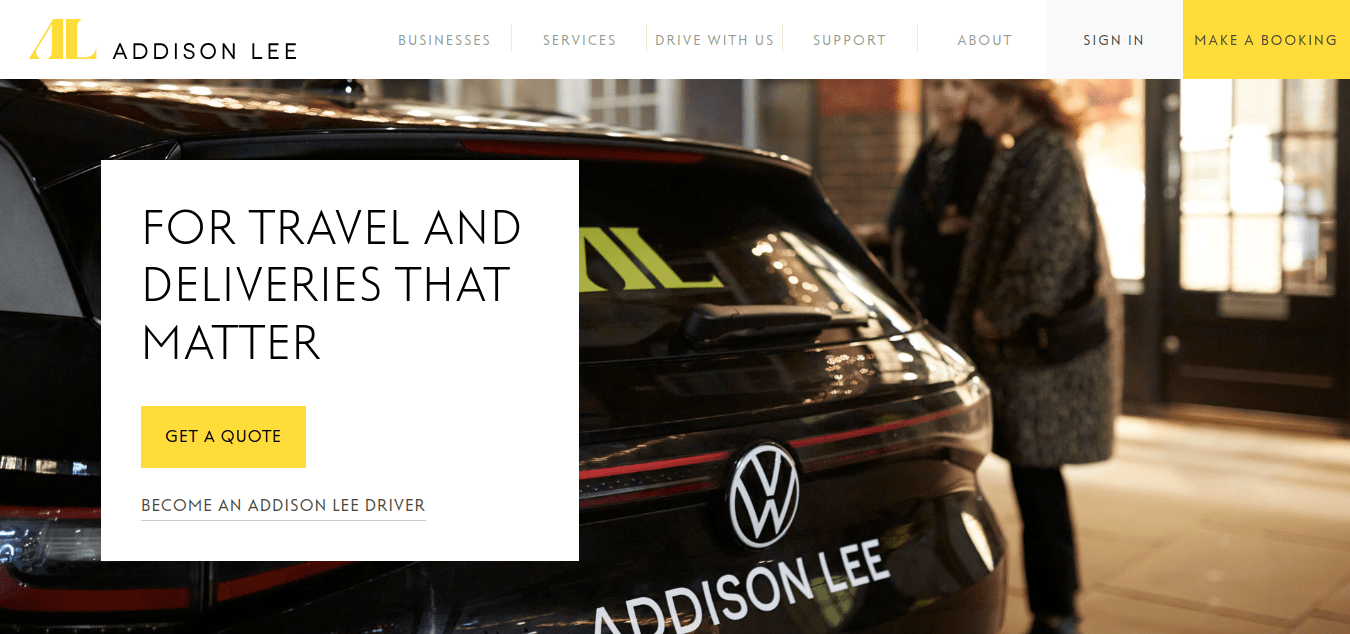The image depicts the homepage of Addison Lee, a company specializing in transportation services. The webpage features a navigational menu at the top with tabs labeled: Businesses, Services, Drive with Us, Support, About, Sign In, and Make a Booking. Dominating the center of the page is a striking photograph of a black Volkswagen vehicle emblazoned with the Addison Lee logo on its side and a large "AL" sticker on the back window. In the background, two women are seen approaching the car, suggesting a pick-up scenario. A prominent white box overlays the image, containing the tagline, "For travel and deliveries that matter." Below the tagline are two actionable buttons: "Get a Quote" for potential customers and "Become an Addison Lee Driver" for prospective drivers. This visually engaging homepage clearly positions Addison Lee as a comprehensive transport service provider, offering easy access for users to book rides or join the company's driver roster.